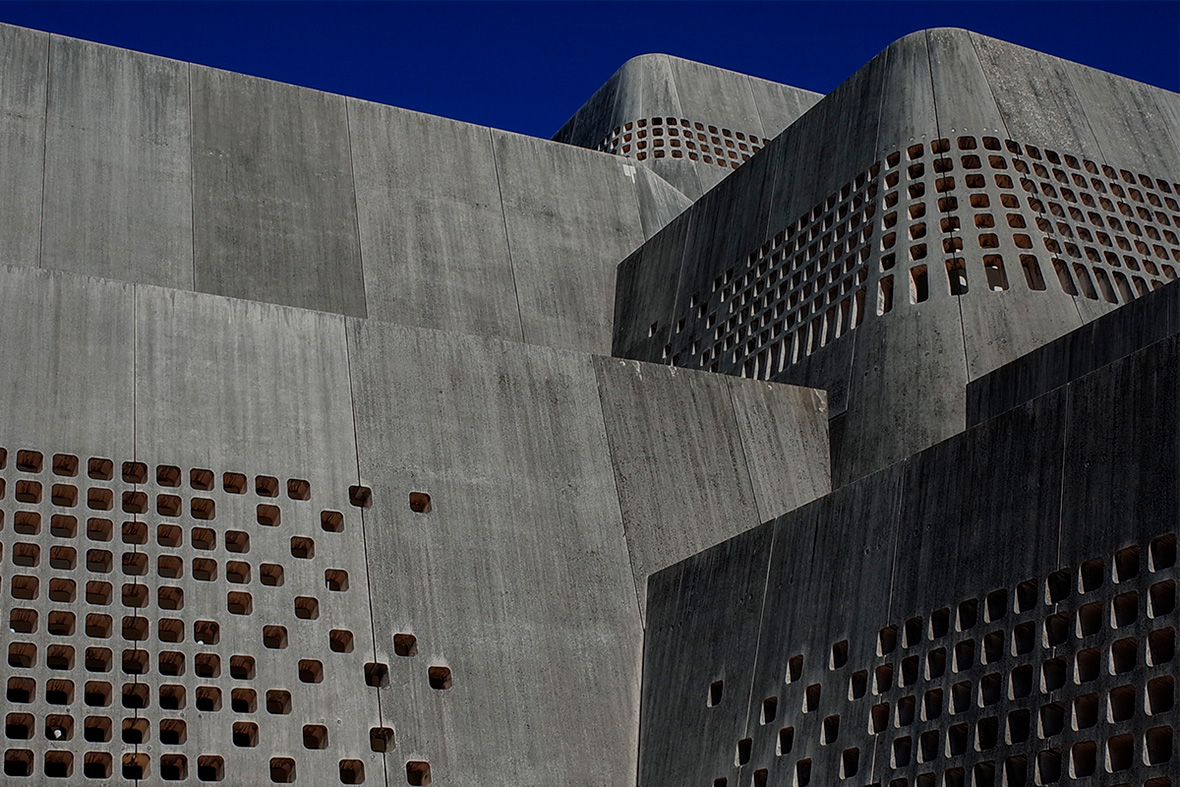The photograph captures the exterior of a vast, multi-leveled building constructed primarily from dark gray cement, creating a foreboding, almost mysterious ambiance. The façade features numerous square-shaped cutouts with curved corners, meticulously arranged in some areas into organized rows and columns, while other sections exhibit a more sporadic pattern. These unusual apertures, too small to be typical windows since they lack any glass, punctuate the building's austere appearance. The structure is composed of wide, rectangular stone sections, subtly streaked in varying shades of gray. The edifice seems to be built in tiers, with each level maintaining the same architectural style. Above, the sky is a clear but dark blue, adding to the enigmatic nature of the scene. The photograph's horizontal alignment emphasizes the expanse of the imposing building, making it the central focus with very little sky visible. The absence of any human presence further intensifies its eerie, almost intimidating vibe, leaving one to ponder its purpose—be it industrial, governmental, or something more clandestine.